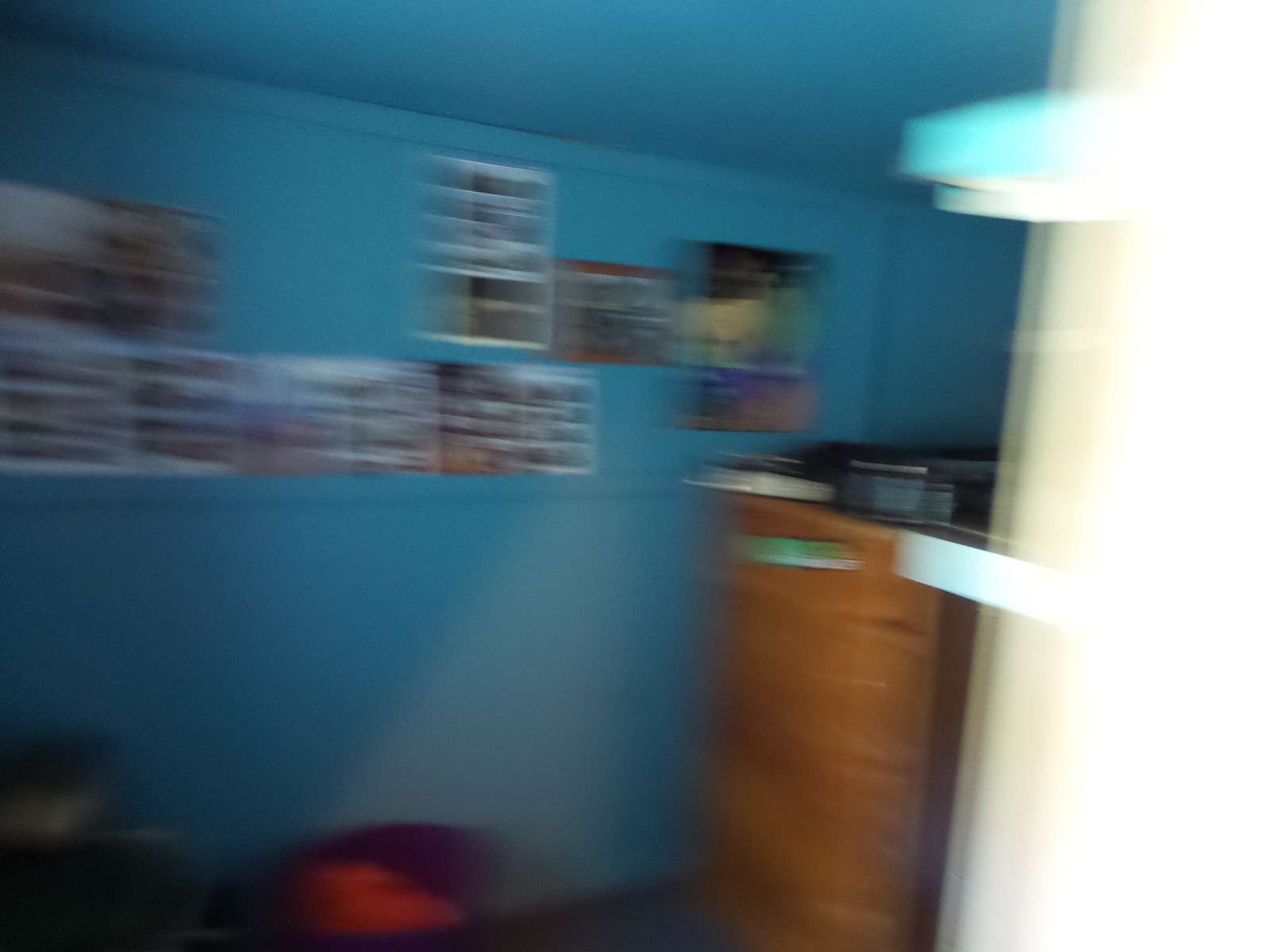This is a very blurry photograph of the interior of a room, characterized by light blue or turquoise painted walls and ceiling. The right side of the room features a light brown, wood-paneled piece of furniture that could be either a desk, a chest of drawers, or a pedestal, holding a pile of white and black items, possibly stacks of books or other debris. The walls are adorned with numerous busy-looking rectangular and square-shaped posters or photo prints, some of which might be collages, framed images, or even action figures still in their packaging. Visible in the bottom right corner is a purple, oval-shaped bucket with a red object inside. A white doorway is also discernible on the right side of the image.